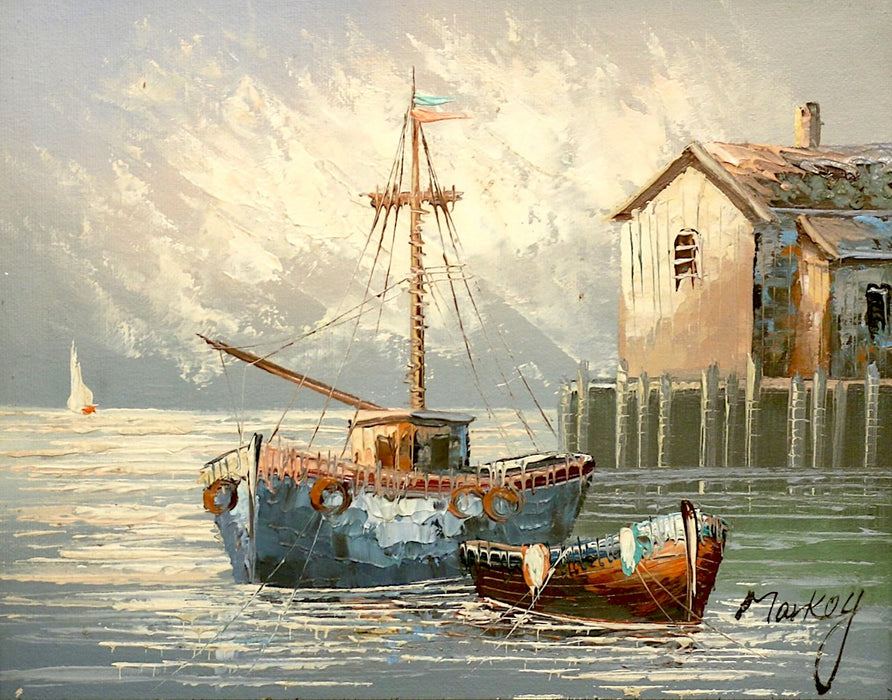This detailed oil painting by M. A. R. K. O. Y. Marquois, signed by the artist, captures a maritime scene with thick, expressive brushstrokes. The composition is centered around a large vessel with substantial rigging but no sails raised. The ship's hull is predominantly gray, green, and white, with brownish life buoys hanging from its side. Adorning the vessel, two pennants flutter in the wind—a sharp pointed light blue one above a slightly larger, more brown pennant. In the background, towards the right, stands a dilapidated, brown house, adding a sense of history and wear to the overall scene. The rough, textural quality of the paint applied to specific areas, especially the boat, enhances the painting's depth and realism.